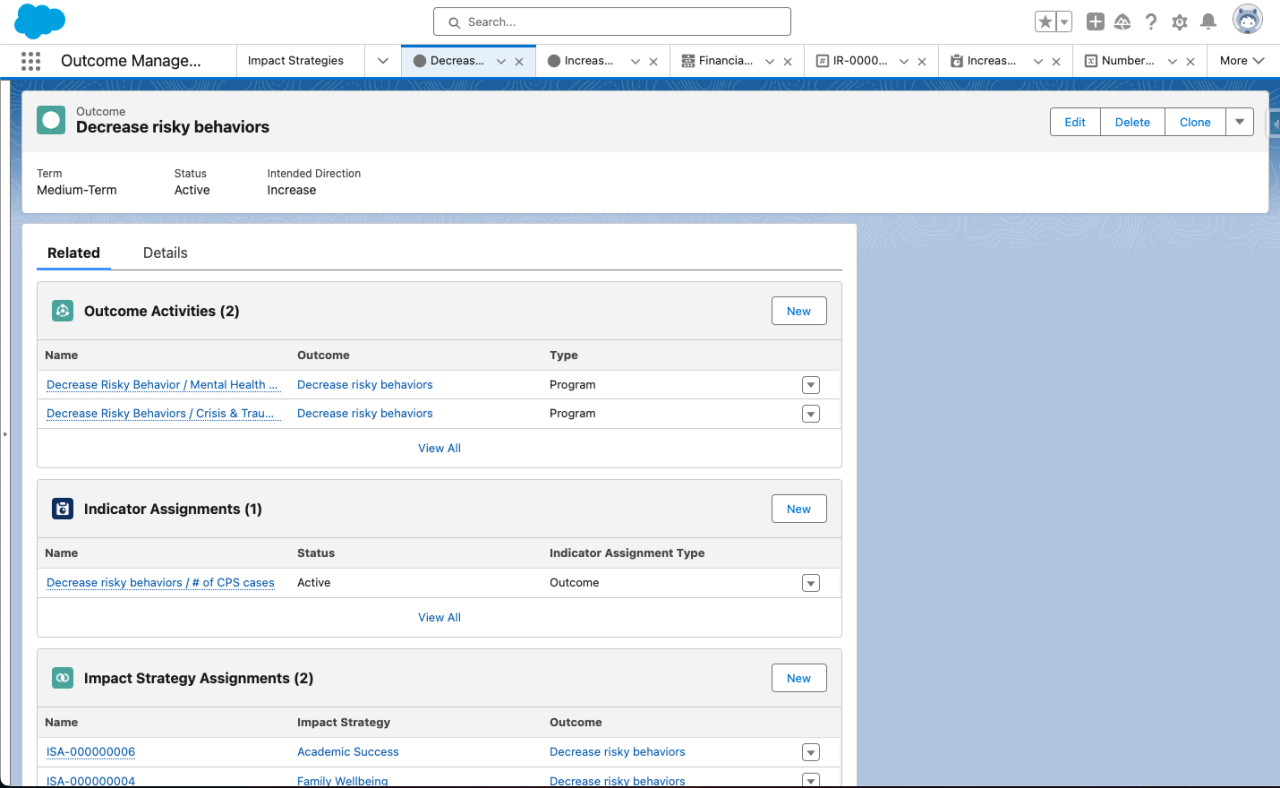This screenshot depicts a webpage that appears to be a type of software likely used by IT professionals, possibly associated with Salesforce given the blue cloud icon in the upper left corner, resembling the Salesforce logo. The header section has a white background and features several navigational items from left to right, including "Outcome Manage," indicated by three dots, suggesting additional options for a manager perhaps. Other visible items include "Impact Strategies," "Decrease," "Increase," and "Financial," along with a dropdown menu labeled IR-1000 or I-000.

Below the header, the overall page background is light blue, featuring a white rectangular section stretching across the screen. The top part of this rectangle has a very light gray background, displaying bold text that reads "Decrease Risky Behaviors." The text layout underneath is organized into three columns labeled "Term," "Status," and "Intended Direction." The entries read as follows: under "Term," it says "Medium Term"; under "Status," it says "Active"; and under "Intended Direction," it says "Increase."

Further down, there is another rectangle, though this one does not span completely to the right. On its right side, a blue border is visible. This section is also organized into a series of columns with headers. The primary header is "Related," followed by sub-headers "Outcome Activities (2)," "Indicator Assignments (1)," and "Impact Strategy Assignments (2)."